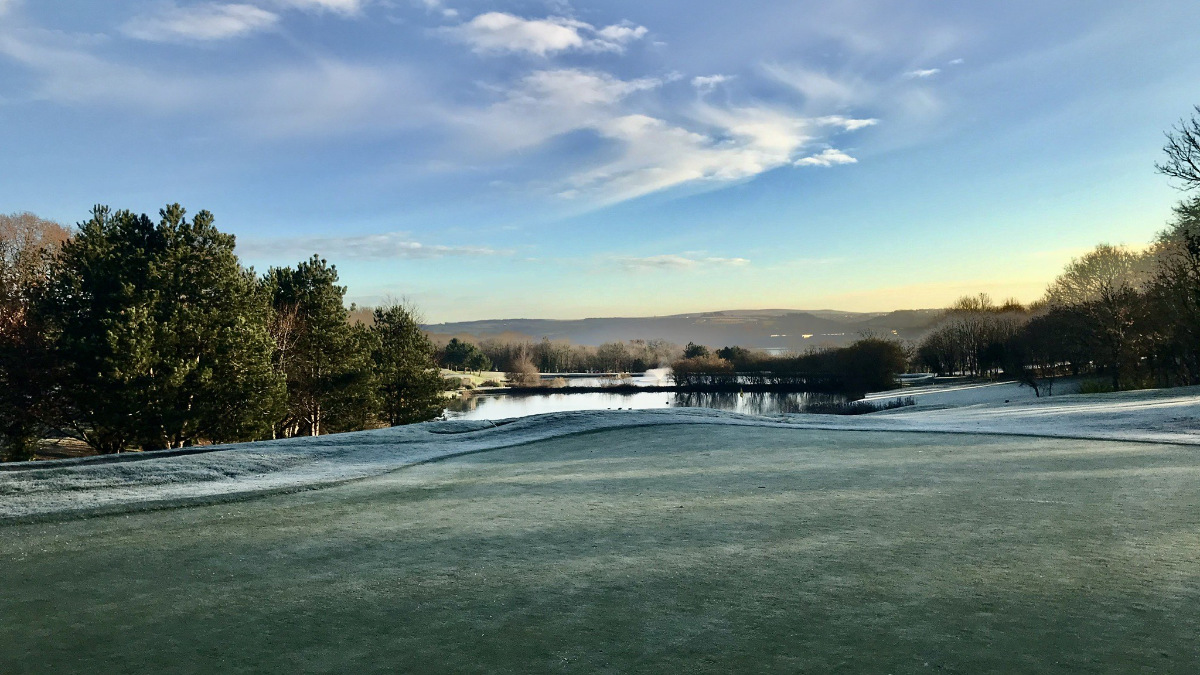This outdoor photo captures a serene landscape with a meticulously maintained grassy area in the foreground, indicative of a golf course, given the vibrant green and evenly trimmed turf. The scene is beautifully lit, suggesting either sunrise or sunset, as the sky transitions from a light tan-yellow at the horizon to a vivid blue. Wispy white clouds are scattered throughout the sky, enhancing the picturesque quality of the scene.

In the mid-ground, a decent-sized body of water, possibly a lake or pond, is centered. This lake appears to be traversed by a causeway, adding an element of human interaction to the natural backdrop. Flanking the water, clusters and rows of mature green trees are positioned on both the left and right, where their reflections can be seen mirrored in the calm water. Some trees' trunks are visible, adding shades of brown to the predominantly green scenery.

As the view extends into the distance, gentle blue hills roll into the horizon, giving way to the vast, bright blue sky overhead. The sky's coloration gently shifts from an orange hue near the horizon to a deeper blue, accentuated by the diffusion of white clouds that appear to ride along the mountain tops.